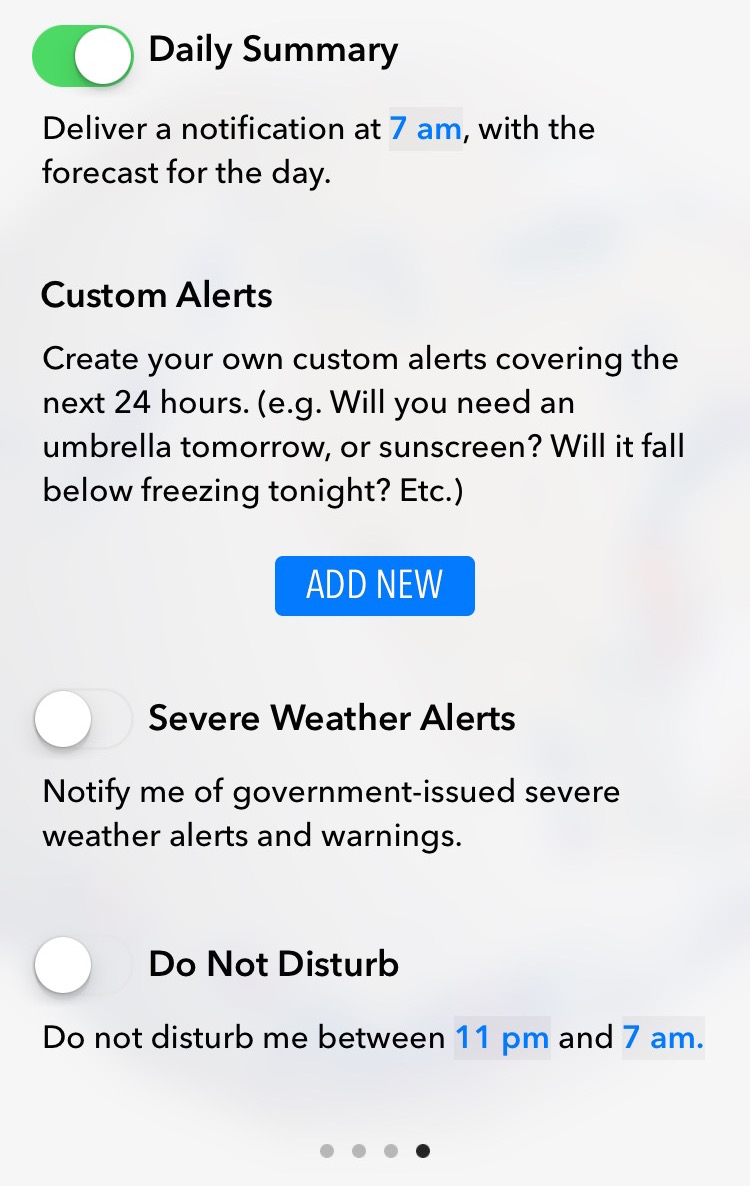The image depicts a detailed view of a weather alert settings screen. At the top left, there is a green toggle switch that is turned on. Next to it, in black font, is the title "Daily Summary." Directly below, in smaller black font, the text reads: "Deliver a notification at 7 AM with the forecast for the day." The "7 AM" is highlighted in blue font and enclosed within a light gray square.

Following this section is a bold black font title labeled "Custom Alert." The accompanying description in smaller black font states: "Create your own custom alerts covering the next 24 hours (e.g., will you need an umbrella tomorrow or sunscreen? Will it fall below freezing tonight?)." Below this description is an "Add New" button.

Further down, two additional settings are displayed: "Severe Weather Alerts," which is toggled off, and "Do Not Disturb," also toggled off.